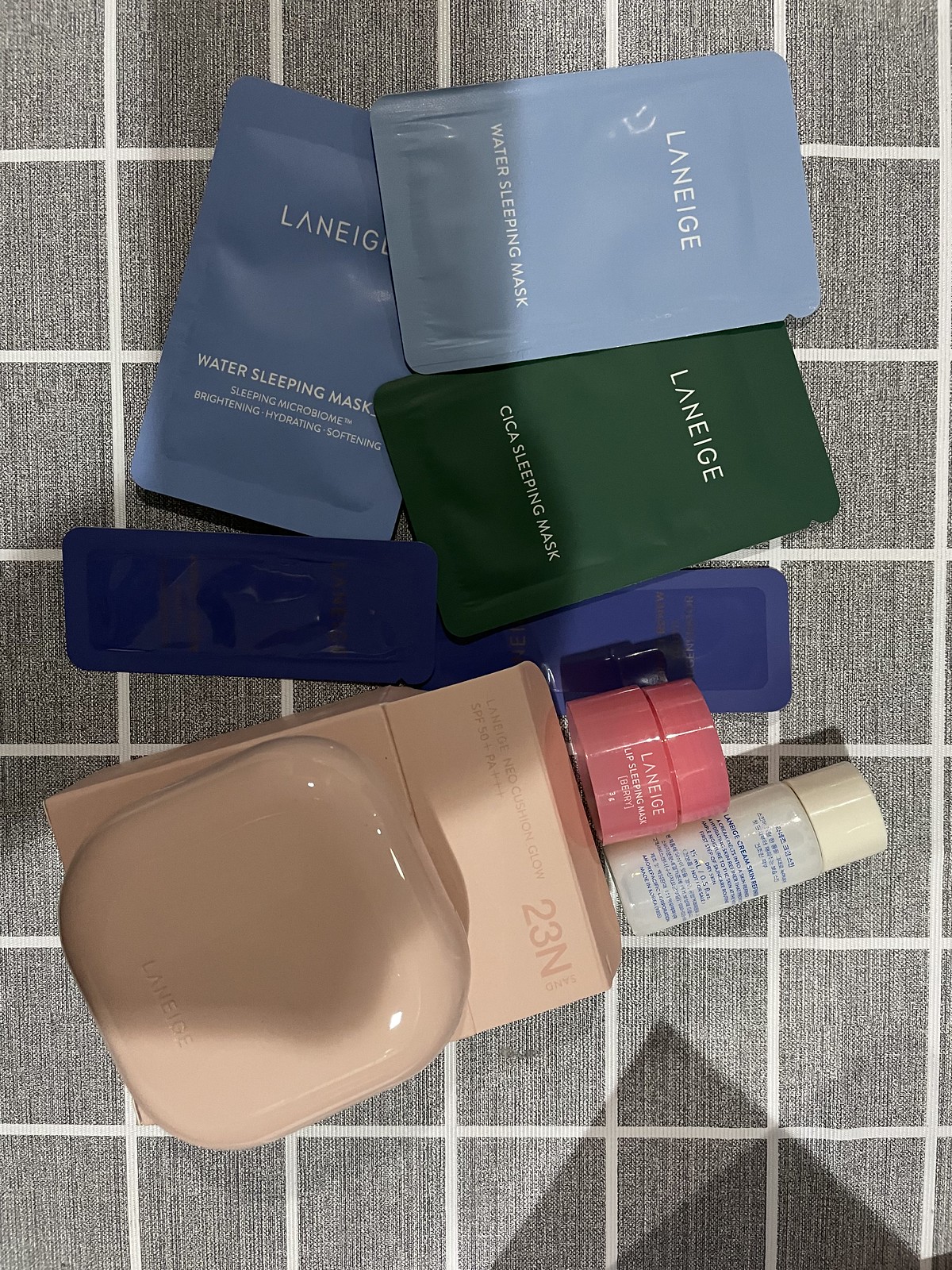This image, captured indoors with a standard camera, presents an array of skincare and cosmetic products arranged on a flat surface. Rotating the image 90 degrees to the left would significantly improve readability and visibility of the items.

At the top of the image, there are two disposable packages from the brand Laneige (spelled L-A-N-E-I-G-E). The left package is a light grayish-blue and labeled "Water Sleeping Mask," while the right package is hunter green and labeled "Cica Sleeping Mask." Below these, closer to the bottom, another Laneige "Water Sleeping Mask" package is visible, distinguished by a darker blue color and additional print.

Towards the middle of the image, two tubes containing facial moisturizer or another liquid skincare product are present. Adjacent to these is a peach-colored box featuring a cube-like shape on top, with "23N" printed on it.

Centrally positioned amidst these items is a blue, rectangular piece of plastic, adding a contrasting visual element to the composition.